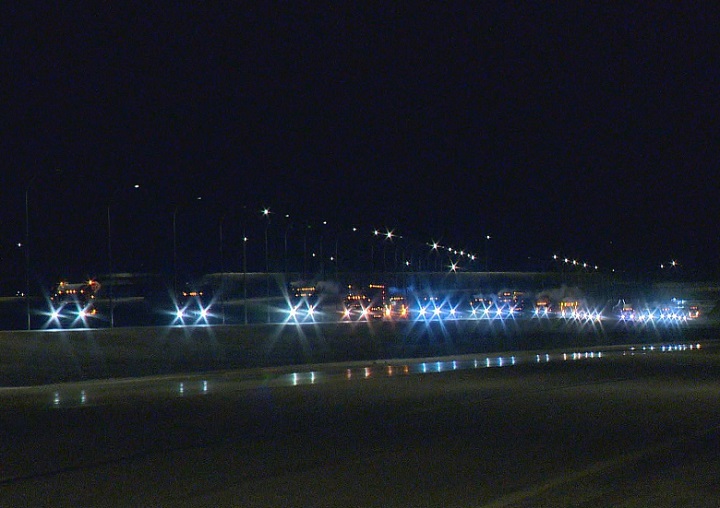The photograph captures a nighttime scene on a wet divided highway with a convoy of 18-wheeler trucks heading toward the camera. The photographer is positioned next to an empty lane, observing the oncoming traffic from the opposite side. The trucks, numbering between 20 to 25, have headlights that vary from warm incandescent yellow to cool blue halogen or LED, creating a star-like distortion due to water droplets in the air. Rows of street lamps along the highway cast a limited illumination, reflecting off the wet pavement and enhancing the sense of darkness in the black sky. The backdrop is solid black, with only the glowing headlights and faint streetlights piercing through the night. The surrounding area shows a slight border of grass and another road, giving depth to the image. The headlights' reflections in the wet asphalt amplify the surreal and almost poetic atmosphere of this nocturnal highway scene.